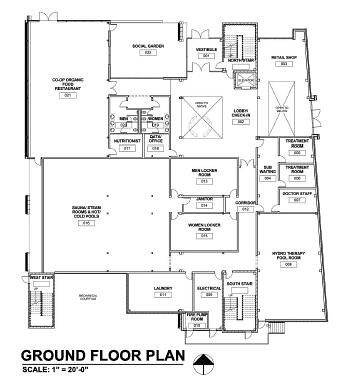Floor plan analysis of a multi-story commercial building, rendered at a scale of 1 inch equals 20 feet. The plan features several rooms, suggesting an expansive layout indicative of an office building or another non-residential facility. 

Key elements include:
- Three separate staircases
- An elevator shaft
- Multiple entrances, totaling at least four
- A room labeled "Electrical"

Although the text is too small to decipher clearly, the use of structural elements and the number of rooms implies a sophisticated and sizable commercial space rather than a residential property.